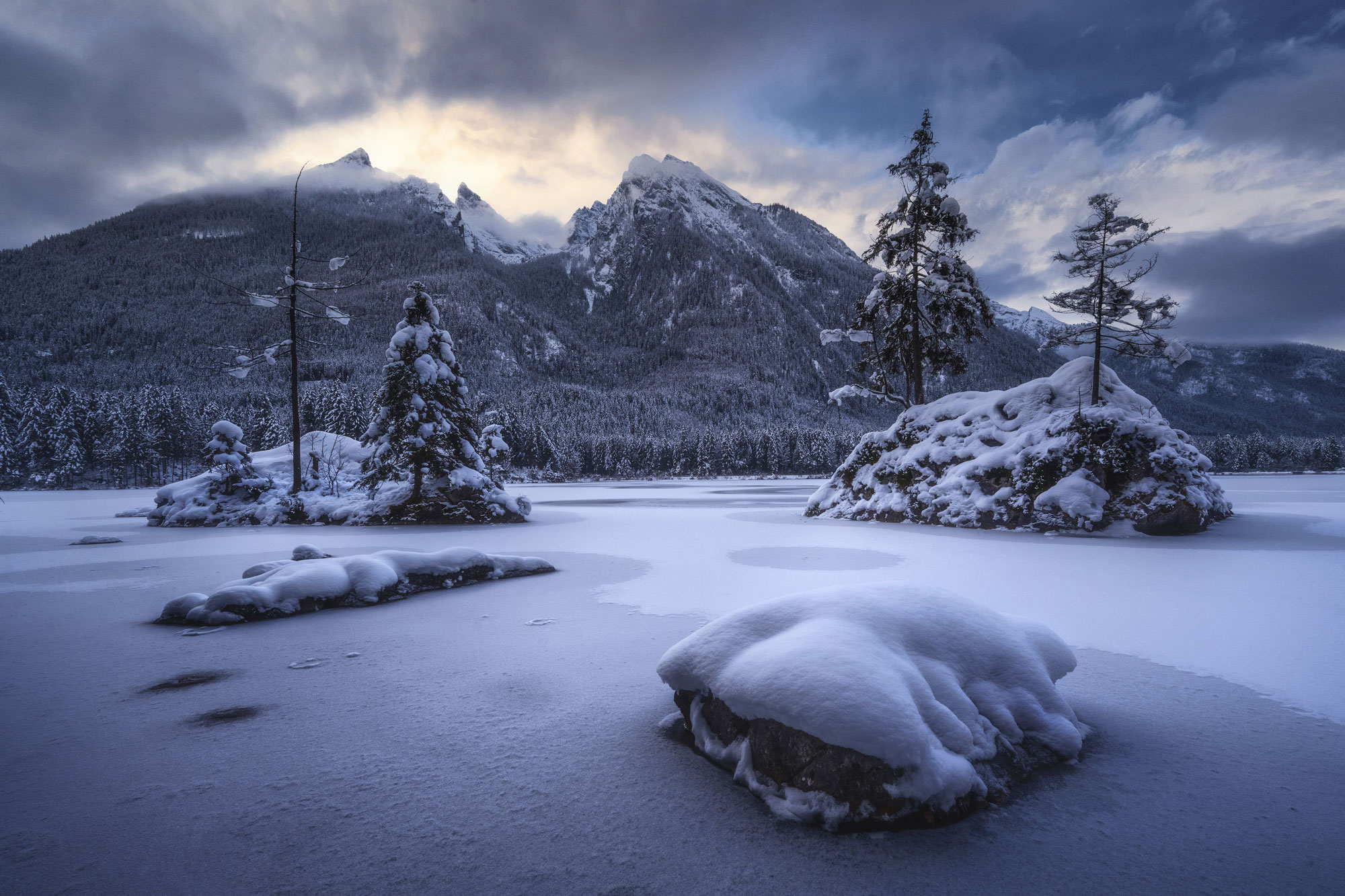This outdoor daytime photograph captures a breathtaking winter wilderness scene, dominated by a looming storm sky that transitions from dark thunderous clouds at the top to lighter blues and grays below. A majestic mountain landscape with snow-capped peaks stretches across the background, with the tallest peak piercing the cloud layer on the left side. In front of the mountains lies a frozen lake, its surface untouched and smooth, reflecting the icy stillness of the scene. The lake is dotted with several rocks, some of which emerge as small islands. The largest rock, situated at the center, is blanketed by approximately 4-5 inches of snow. To the right, a rock island supports two resilient trees, while the left rock has one living tree and another that appears lifeless, possibly charred. Snow-laden trees, their branches bowed under the weight, frame the foreground and scatter throughout the landscape. The entire vista conveys an awe-inspiring sense of tranquility and the harsh beauty of winter.